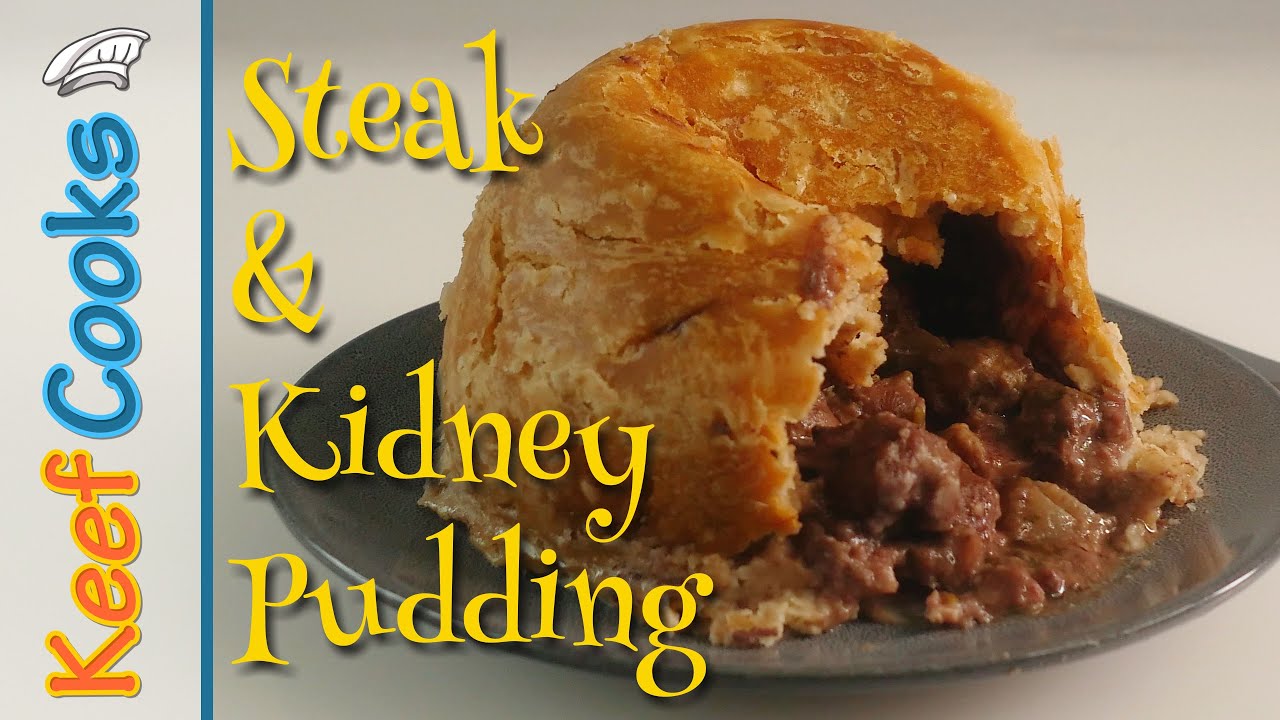The cover image for the article featured on the web prominently displays a large photo of a dish labeled "Steak and Kidney Pudding." The dish is showcased on a dark gray plate, with the golden brown crust of the pudding revealing a darker reddish-brown meat filling through a cut in the pastry. To the left of the image, text runs vertically from bottom to top, spelling out "Keef Cooks" in a fun, comic-style font with "Keef" in orange and "cooks" in blue, topped with a chef's hat symbol above the 'S'. The background of the overall layout is an off-white hue, subtly blending with the plate and putting a strong emphasis on the richly colored steak and kidney pudding. The pudding appears moist and flaky, adding to its appealing presentation as the main highlight of the image.